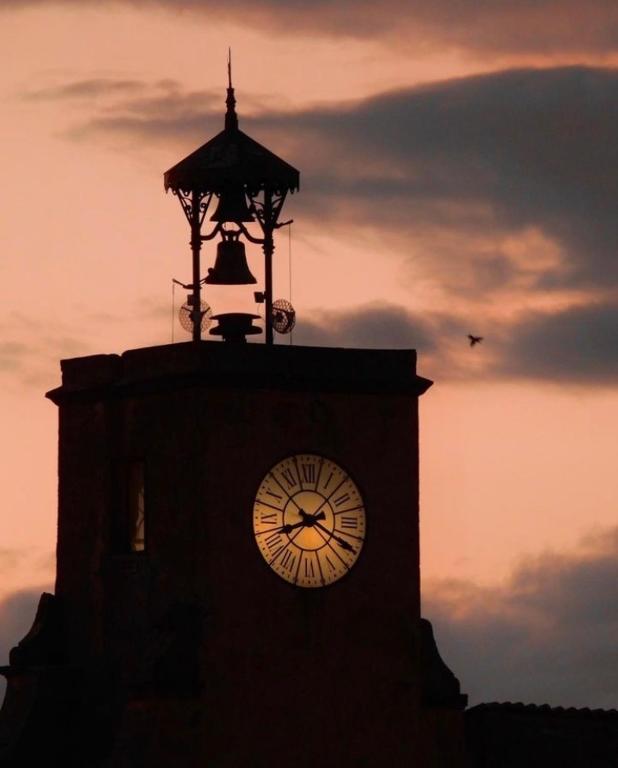The image captures a clock tower at dusk, against a picturesque sky where pink hues mingle with dark and light-colored clouds, indicating the sun has already set. The face of the clock, which displays Roman numerals and shows the time as 8:20, stands out vividly as it is illuminated against the shadowed tower. Above the clock face, a bell is nestled under a pointed A-frame roof, with ropes attached, suggesting it can be rung manually. A bird, almost silhouetted, flies near the side of the tower, adding a serene touch to the composition. The overall scene appears tranquil and could be reminiscent of a European setting.